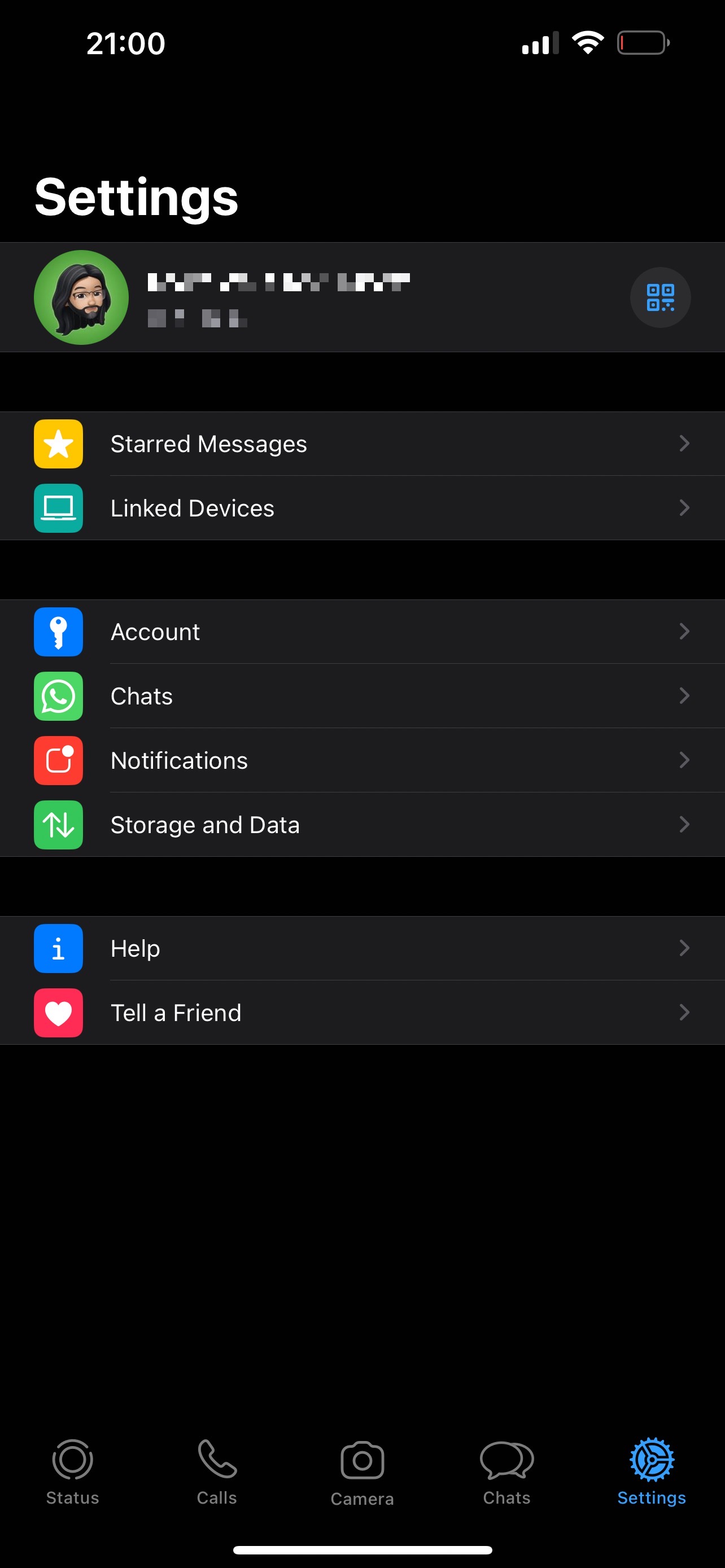This image is a screenshot of a WhatsApp settings page on a smartphone. The background is black, typical for a dark mode setting. At the top of the screen, the time is displayed as 21:00 in white text. The status bar also shows a network signal icon with an incomplete signal, a fully filled Wi-Fi icon, and a nearly depleted battery icon indicated by its red color.

Below the status bar, the word "Settings" is prominently written in white text. Directly beneath is a profile section with a dark grey background. This section includes a circular profile picture frame containing an image of a cartoon person on a green background. The user's name is blurred out in white.

The main menu lists various options in white text: "Account," "Chats," "Notifications," "Storage and data," "Help," and "Tell a Friend." Each option is accompanied by its respective icon. 

At the bottom of the screen, a navigation bar shows various menu icons typical of WhatsApp. These include icons for "Status", "Calls", "Camera", "Chats", and the currently selected "Settings," which is highlighted in blue text with a corresponding blue icon. The other menu items remain in grey. This detailed layout confirms that the screenshot is indeed from the WhatsApp application.